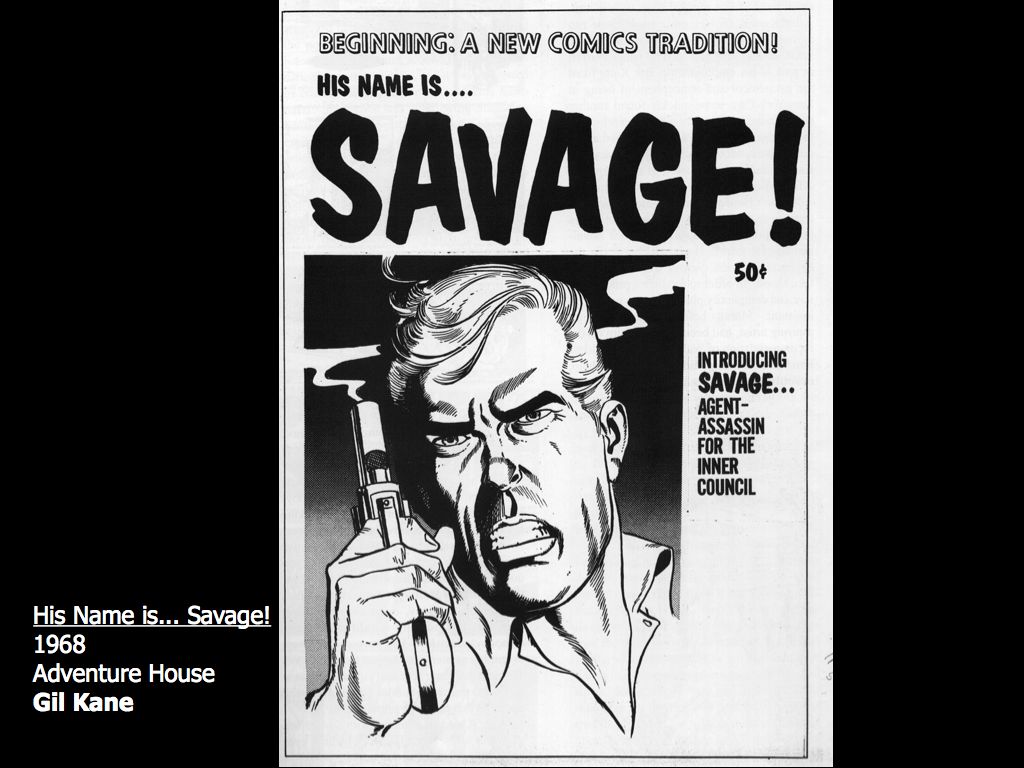This image is a vintage black-and-white comic book cover set against a landscape-oriented black background with black side panels. The comic book itself, centered in portrait orientation, features a white background with prominent black lettering. At the top, it reads, "Beginning: A New Comics Tradition!" followed by "His Name Is..." in smaller black text and "Savage!" in bold, large letters. Priced at 50 cents, the cover also announces, "Introducing Savage, Agent-Assassin for the Inner Council."

The focal point of the cover is a detailed, line-art illustration of Savage—a close-up of a man with a wavy, unkempt hairstyle and an intense, gritting-teeth expression. He holds a revolver in his right hand, pointed upwards with smoke trailing from the barrel behind his head. Savage is depicted wearing a white polo or button-up shirt.

In the bottom left, beneath the main comic book image, there's another panel with text that reads, "His Name Is Savage, 1968, Adventure House," and in bold, "Gil Kane," presumably attributing authorship or illustration to Gil Kane.